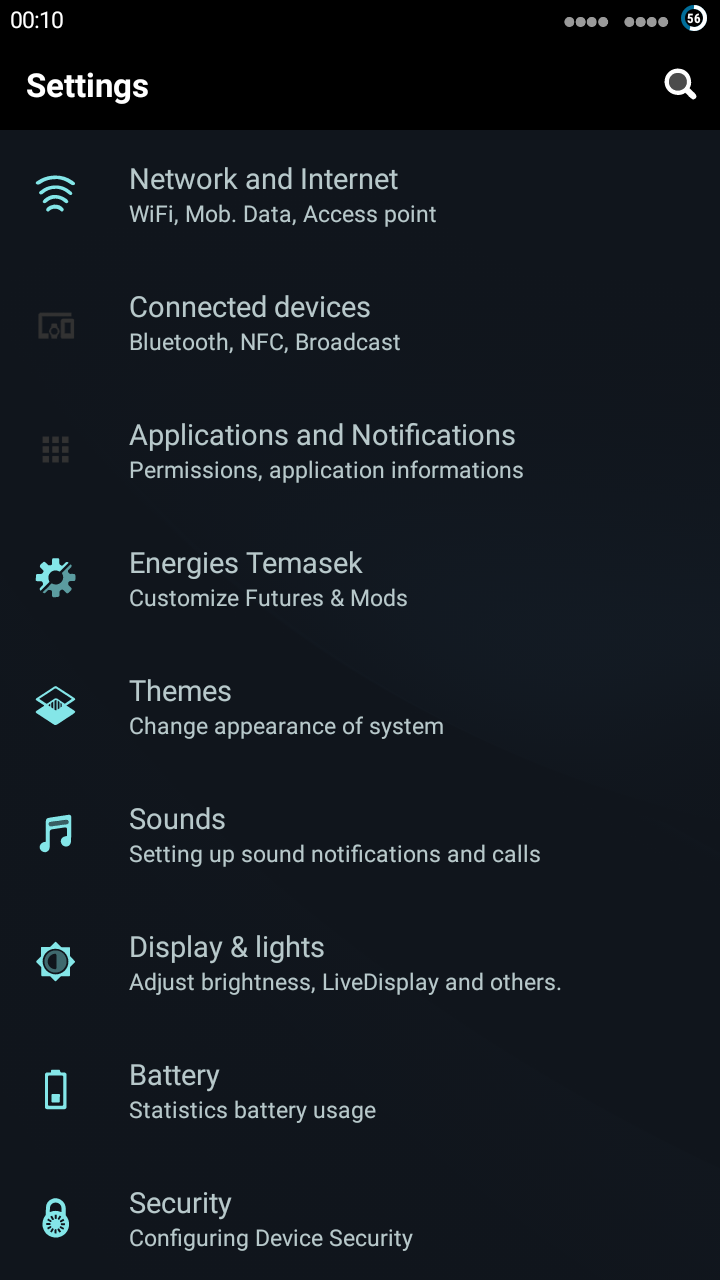A high-resolution screenshot captured from a smartphone interface is displayed. In the top left corner, the time reads "00:10", followed by a signal strength indicator composed of four filled dots and an additional four unfilled dots, suggesting Wi-Fi status. Adjacent to this, within a half-white, half-blue circle, the number "56" is prominently shown, potentially indicating battery percentage or an app notification.

Beneath this bar lies the main interface, starting with "Settings" in bold white text on the left, accompanied by a magnifying glass icon for search functionality on the right. Below this heading, a series of categorized settings are listed vertically, each preceded by representative icons.

1. **Network & Internet** - Connectivity options.
2. **Connected Devices** - Includes Bluetooth, NFC, and related broadcast settings.
3. **Apps & Notifications** - Manages permissions and app-specific information.
4. **Energies & Temasek** - Custom features and modifications.
5. **Themes** - Options to change system appearance.
6. **Sound** - Adjustments for sound notifications and call settings.
7. **Display & Lights** - Controls for brightness, live display, and additional settings.
8. **Battery** - Statistics and usage information.
9. **Security** - Configures device security settings.

Each category is succinctly described and paired with intuitive icons, such as a musical note next to Sound settings and a lock symbol beside Security, enhancing the visual layout and ease of navigation.